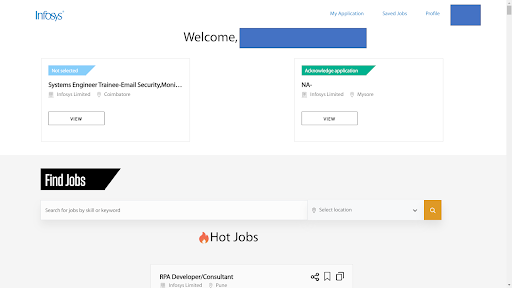Detailed Caption: 

The image depicts a job application website interface designed for users to search and apply for jobs. At the top of the page, there is a blue navigation bar featuring options such as "My Application," "Saved Jobs," and "Profile." The user is currently logged in, but their personal information is obscured by a blue square for privacy. 

Centrally, the page displays a greeting message that reads, "Welcome," likely followed by the user's name, which is also covered by a blue square to protect their identity. The left-hand side of the interface shows the name "Infosys," indicating the company or the website's host. Below this, there is a job listing for a "Systems Engineer Trainee" focusing on "Email Security," with a status of "Not Selected."

On the right-hand side, there's a section titled "Acknowledge Application," which likely allows the user to view or acknowledge their job application status. 

Further down, there is a prominent "Find Jobs" button in white text against a black background. Adjacent to this is a functional search bar where users can input job titles and select a preferred location. 

Beneath the search bar, there is a brightly illustrated "Hot Jobs" section, highlighted with a flame icon. At the bottom of the interface, a listing for "FPA Developer Consultant" is visible, accompanied by various icons enabling users to share or save the job post or the webpage.